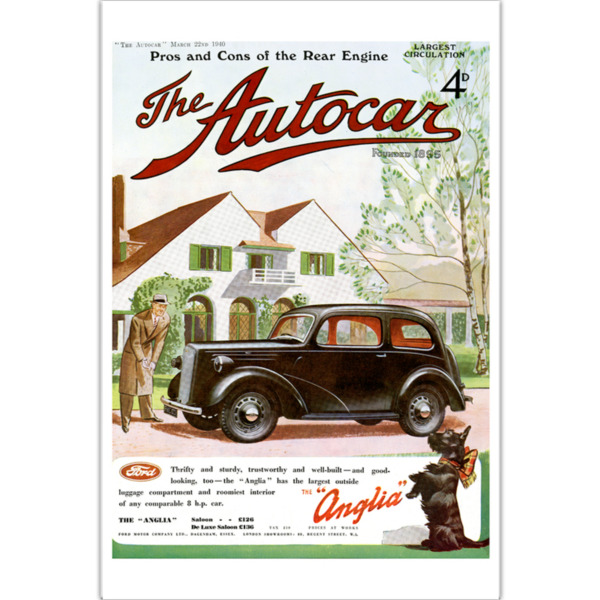This vintage color advertisement, likely from a magazine, showcases a sleek, black Ford car with a red interior in front of a large, traditional suburban home featuring green windows and a balcony. At the top, it reads "Pros and Cons of the Rear Engine" in a nostalgic font, with "The Auto Car" prominently displayed in red cursive. The tagline highlights "Largest in Circulation - Founded 1855." 

In the image, a well-dressed man stands in a brick driveway, examining the Ford vehicle. He wears a brown trench coat and a white and black hat, exuding a stylish early 1900s vibe. On the bottom, the ad includes the Ford logo accompanied by descriptive phrases like "sturdy, trustworthy, and well-built," emphasizing the car's roomy interior and impressive baggage compartment. A small black dog, reminiscent of the canine character from "The Wizard of Oz," adds charm, sitting on its hind legs with a red and yellow plaid bow around its neck.